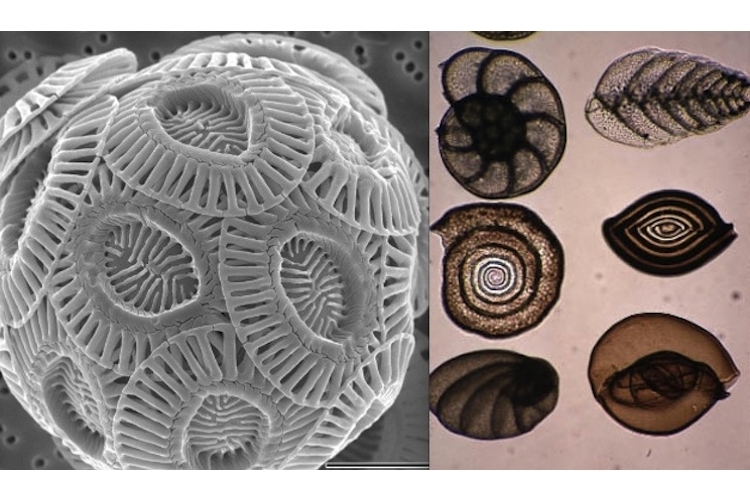This image showcases two distinct, magnified subjects side by side. On the left side, there is a microscopically magnified view of a spherical object resembling a microorganism. This orb appears white and gray and is covered with segmented circular rings that have fingerprint-like fibers within their depressions. The orb also features T-shaped structures protruding from its surface, adding to its intricate, organic appearance. On the right side, arranged in three rows of two, are six seashell-like shapes that look like fossilized specimens. These shells exhibit various forms, including circular, oval, spiral, and leaf shapes, all presented in brown or tan tones against a white background. The shells seem somewhat translucent, allowing internal structures to be visible, and the overall visual suggests an x-ray or thinly cut fossil display.